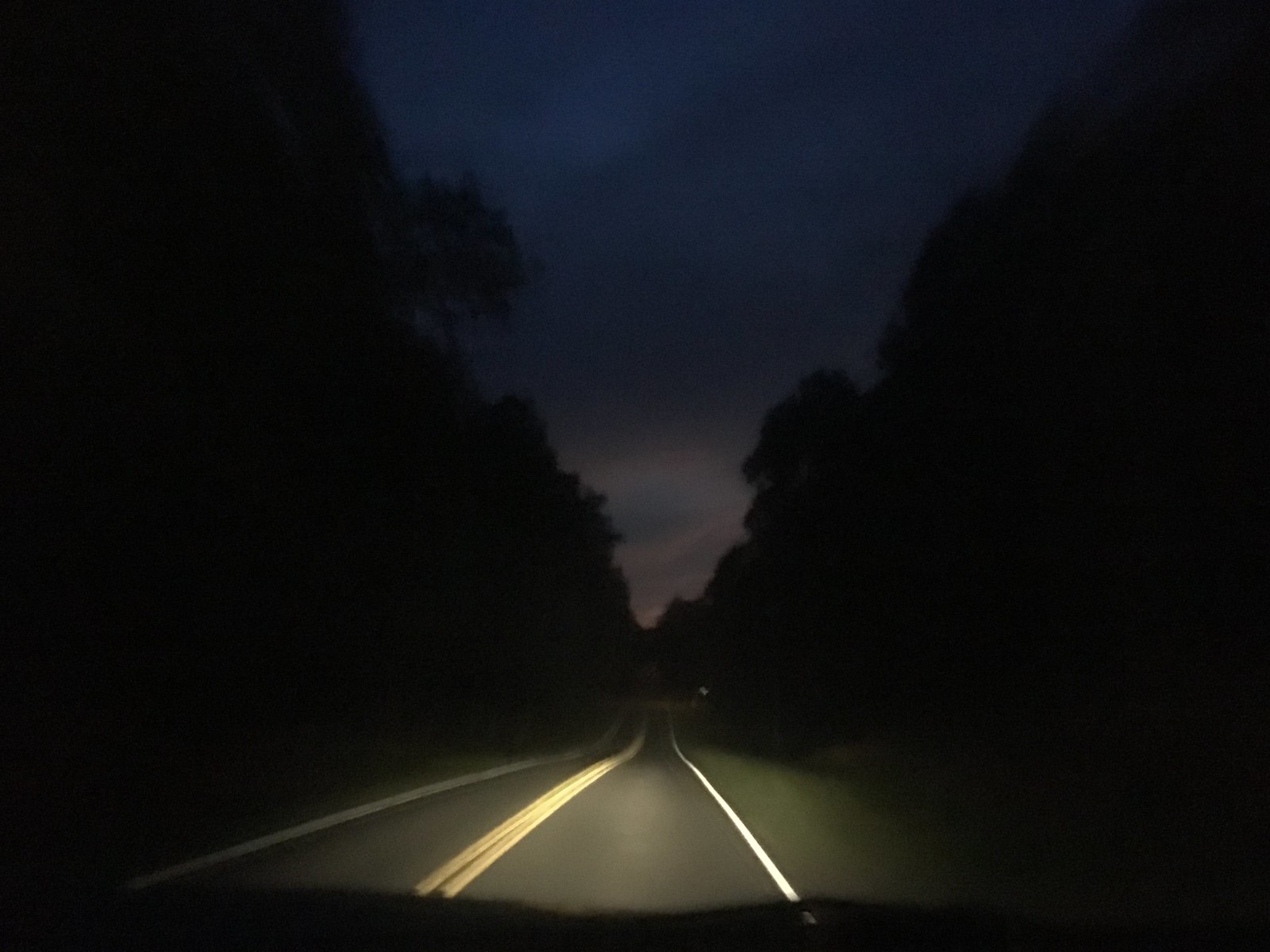A lone driver navigates a bumpy two-lane road under a mesmerizing night sky, adorned with hues of purple, blue, and hints of pink. The journey is flanked by an ominously dark forest line on either side, adding an air of mystery and solitude. The scene invites one to roll down the windows and fully immerse in the tranquil yet eerie surroundings. Despite the road's uneven surface, the allure of the night beckons for a nostalgic nighttime drive filled with starry wonder.